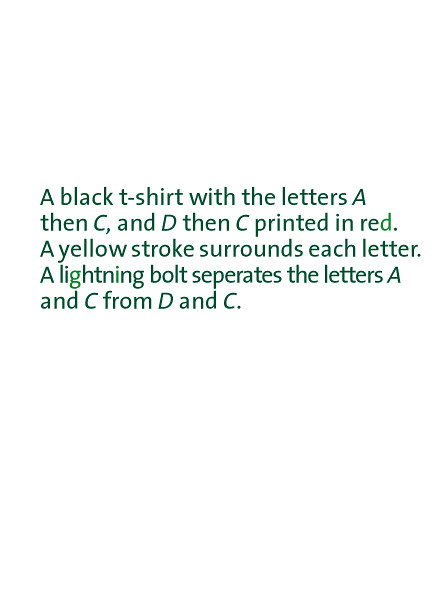The image features centered text against an all-white background. The text describes a black t-shirt adorned with the letters "A," "C," "D," and "C" in red, each letter outlined by a yellow stroke. A lightning bolt separates the sequences "AC" and "DC." The text, written in a sans serif font, is displayed in dark green. This graphic appears to be a description of a logo or design concept for the t-shirt. No other objects or elements are present in the image.